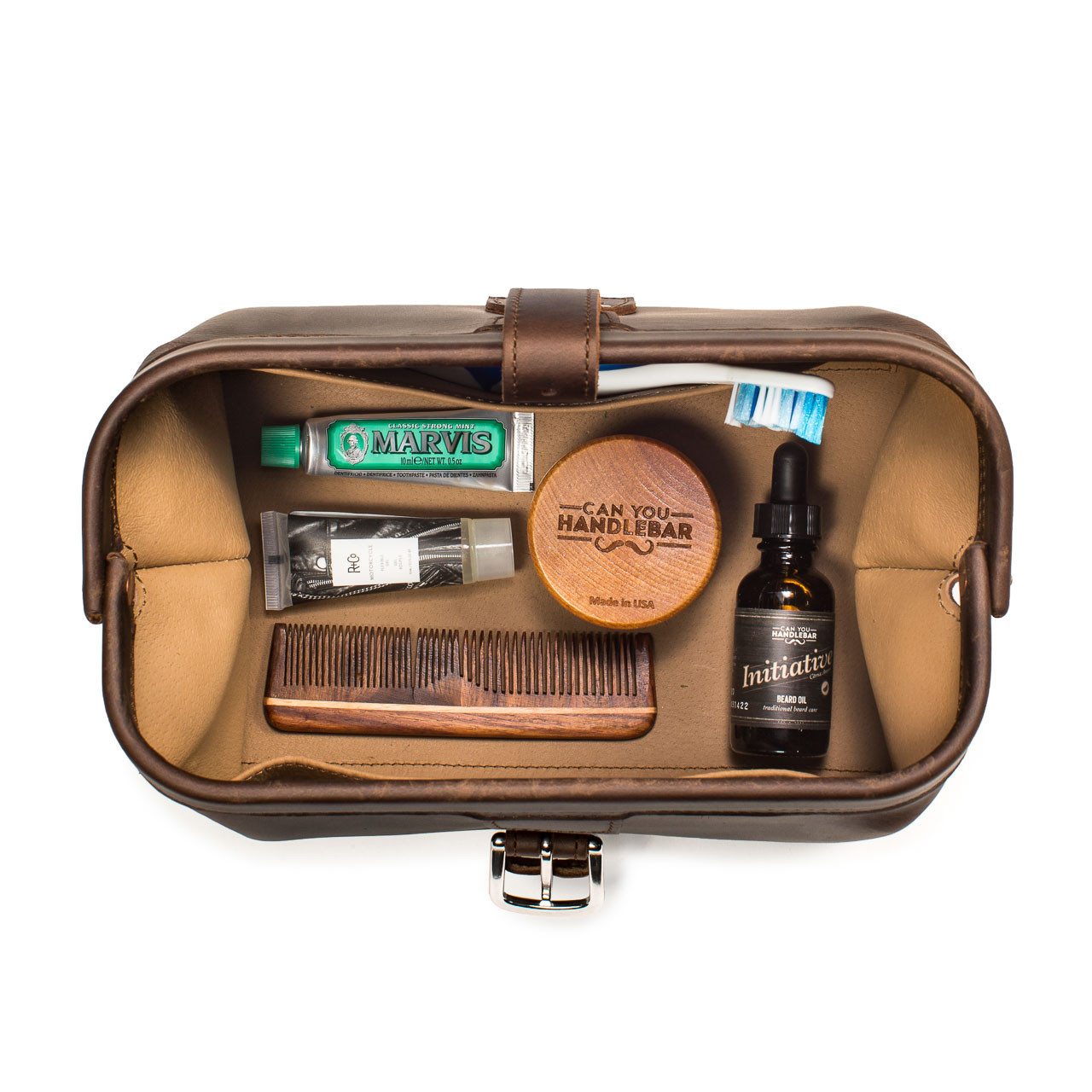This image depicts an open brown leather toiletry bag set against a white background, showcasing its contents from an aerial view. The bag, turned on its side with its open part facing the camera, has a darker brown exterior and a light brown leather interior. It features a top strap in the middle and a buckle hanging from the bottom edge. Inside the bag, a white toothbrush with blue and white bristles is partially visible, protruding from a slot at the top. Below the toothbrush, a green tube labeled "Marvis" with a gray cap stands out, while beneath it, a dark gray tube with a light gray lid and an unreadable white label is positioned. To the left of these tubes lies a brown wooden comb with its teeth facing upwards. Adjacent to the comb on the right is a small brown circular container that appears to say "Can You Handlebar" on its front. Further to the right, a small dark bottle with a black eyedropper-style top and a barely readable label, possibly saying "Imitation" or "Initiative," completes the contents visible inside this meticulously arranged travel bag.